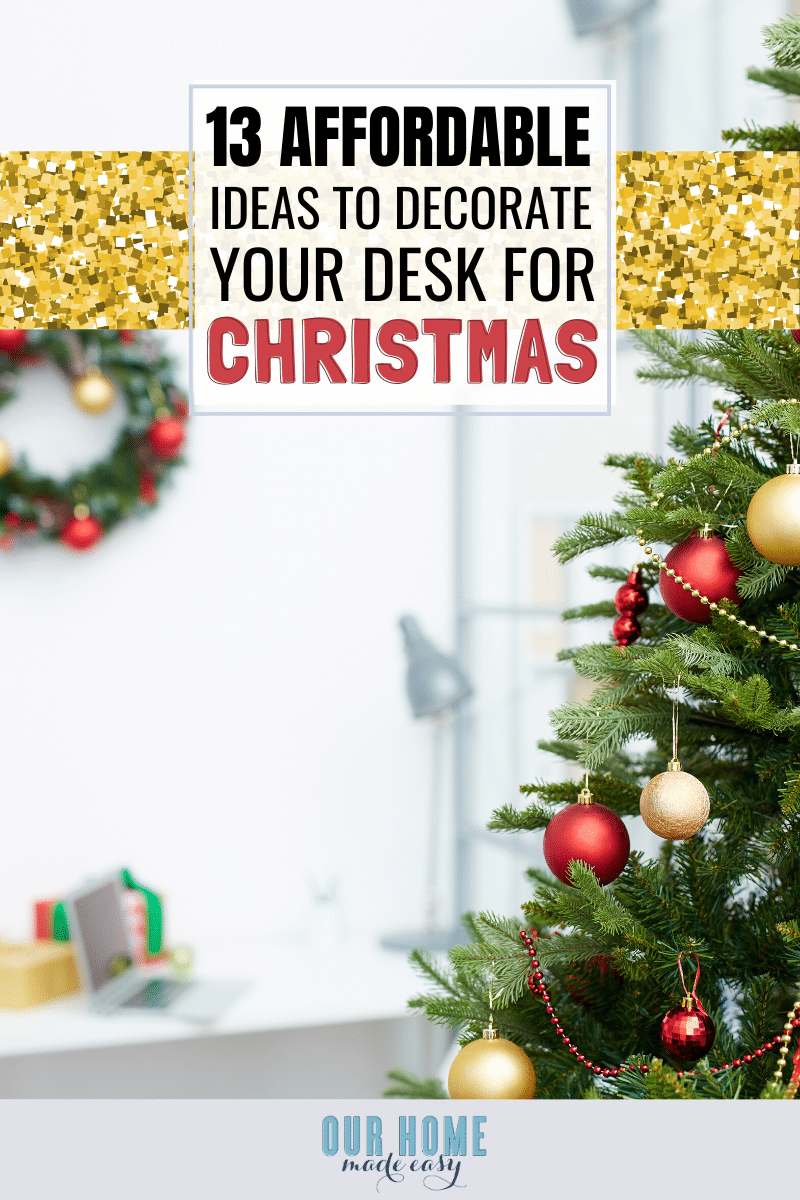This vertical magazine cover features a festive Christmas theme. Dominating the right side is a Christmas tree adorned with red, gold, and silver ornaments, as well as shimmering strands of decorations. The left side highlights a wreath at the top, embellished with colorful red and gold ornaments. The lower section is somewhat blurred, introducing a splash of indistinct colors, possibly from additional decorations or props. A gold glittery banner spans the top of the cover, featuring a white rectangle with the black text, "13 Affordable Ideas to Decorate Your Desk for," and the word "Christmas" prominently in red letters. Below the banner, the publication's title "Our Home" appears in blue letters, accompanied by the black cursive subtitle, "Made Easy." In the background, partial glimpses of what appears to be a window or desk and a silver lamp can be faintly discerned, adding depth to the overall scene.